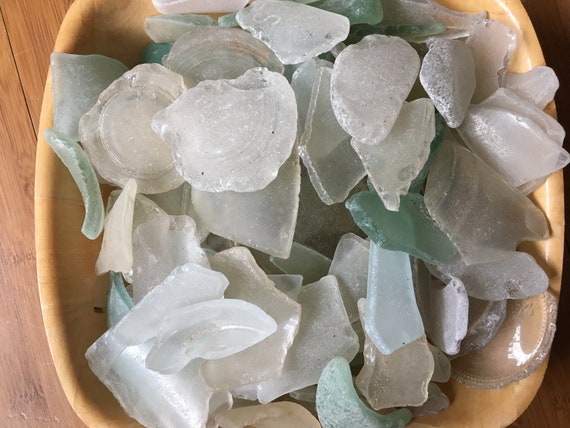This image is a detailed top-down view of a collection of translucent, irregularly shaped sea glass pieces inside a ceramic bowl. The bowl is a rounded square shape and has a rich brown color, enhancing the visual contrast with its contents. The sea glass includes a spectrum of colors such as white, grey, green, and teal, with the teal pieces mostly settled at the bottom. The pieces appear delicate and thin, almost shard-like, with rough edges and a texture that suggests they could easily break if handled roughly. The sea glass is jumbled together, some pieces atop others, creating a layered effect. The bowl rests on a light brown wooden platform, adding a rustic touch to the overall composition.